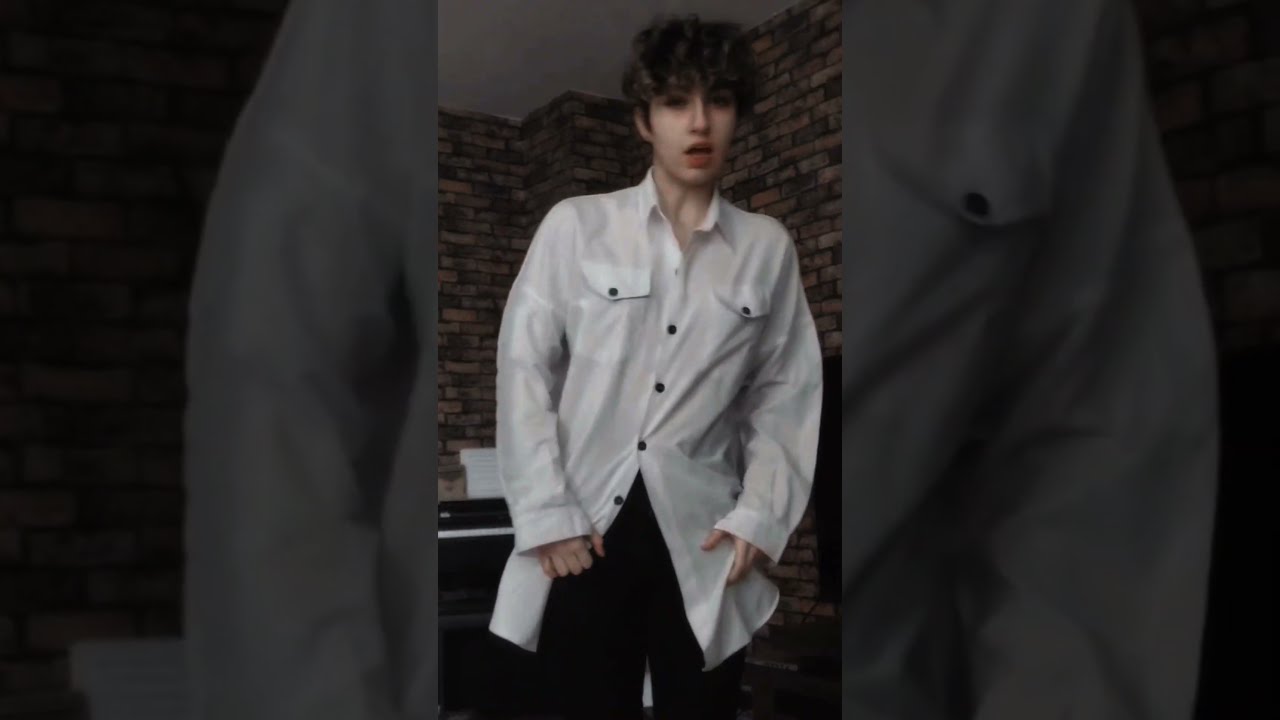The image is a triptych of photographs arranged vertically. The top and bottom panels emphasize the detailing of the subject’s white, long-sleeved shirt with black buttons and pockets, focusing on the right and left arms respectively. These panels feature a dark filter, adding depth and contrast to the image. The middle panel showcases a young man, likely a teenager, with short, wavy brown hair standing against a multi-colored brick wall. He is dressed in the same white shirt—buttoned up only partially—and dark pants. His expression is neutral, with a slightly open mouth, and his hands are visible, appearing as though he is holding his shirt slightly open. The setting includes a detailed brick wall background with shades of dark red, brown, black, and white, as well as hints of a gray ceiling and possibly a piano with sheet music off to one side. The overall lighting in the pictures suggests a dimly lit room during the daytime.